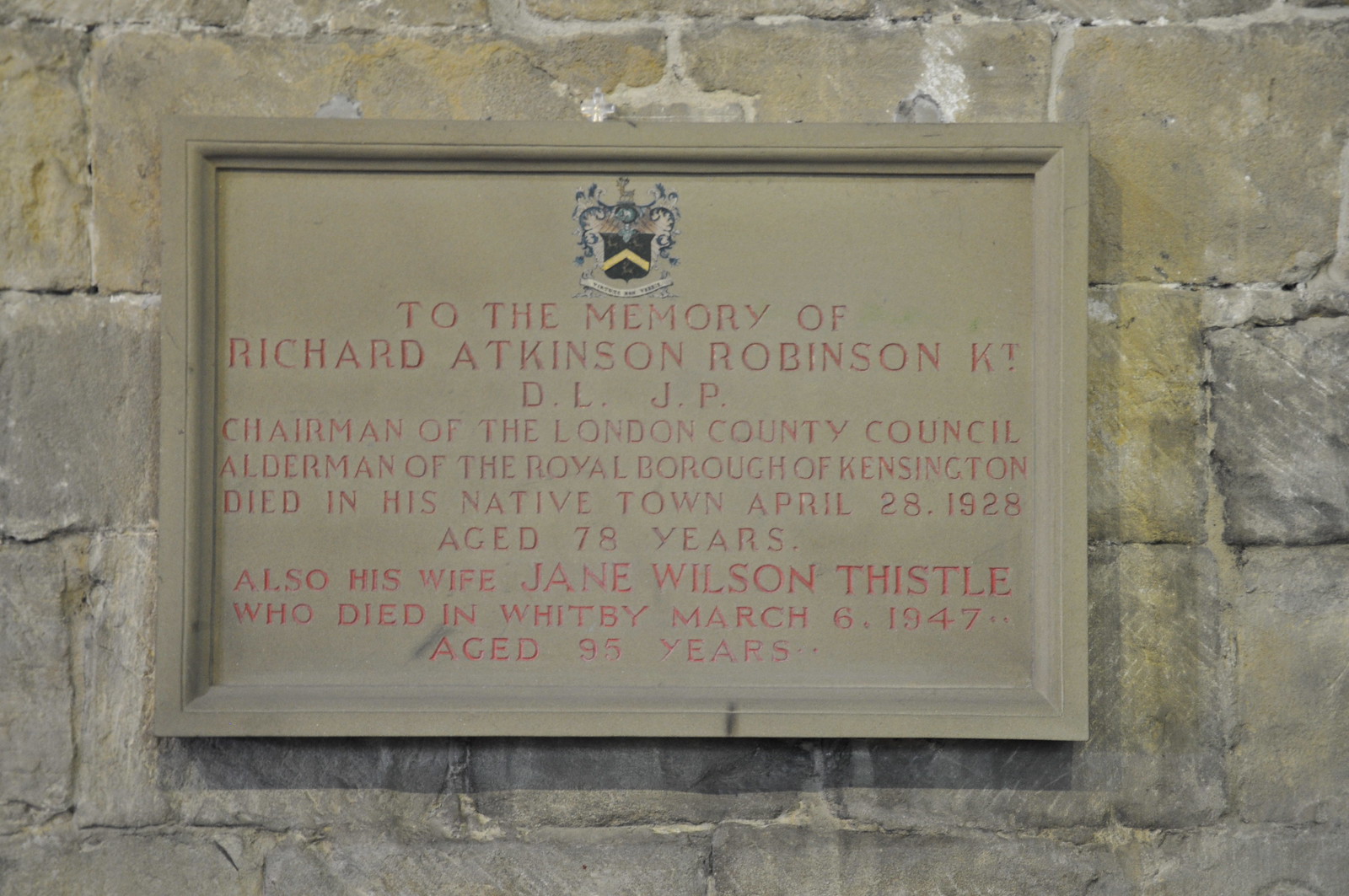In this outdoor photograph, a memorial plaque is mounted on a weathered gray stone wall with patches of yellow discoloration at the top and right sides. The plaque is framed in a material similar in color to the stone wall, possibly beige stone or weathered wood. At the top center of the plaque, there is a black shield with a yellow chevron, bordered by blue and white flowery designs. Below the shield, red text reads: "To the memory of Richard Atkinson Robinson KT DL JP, Chairman of the London County Council, Alderman of the Royal Borough of Kensington, died in his native town April 28, 1928, aged 78 years. Also his wife Jane Wilson Thistle, who died in Whitby March 6, 1947, aged 95 years."